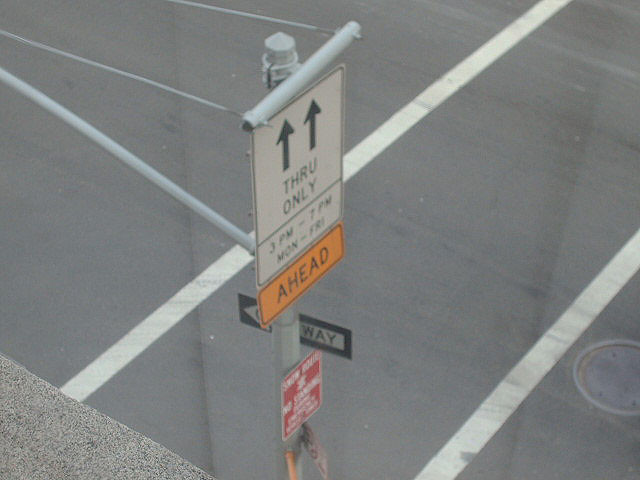This is an aerial view of a street scene taken from a rooftop. In the lower left corner, a flat roof covered with gravel-like roofing material is visible. At the top of the view is a traffic sign displaying several directives. The uppermost sign is white with black text and two arrows pointing straight ahead, indicating "Through Only 3 P.M. to 7 P.M. Monday through Friday." Directly below it is an orange sign bearing the word "Ahead." Beneath this is a red sign, likely a tow-away or no parking sign. To the right of these signs is a one-way sign pointing in the designated direction. The street below is clearly visible, featuring a manhole cover on the far right and a prominently marked crosswalk with white stripes. The street itself is composed of typical gray asphalt.